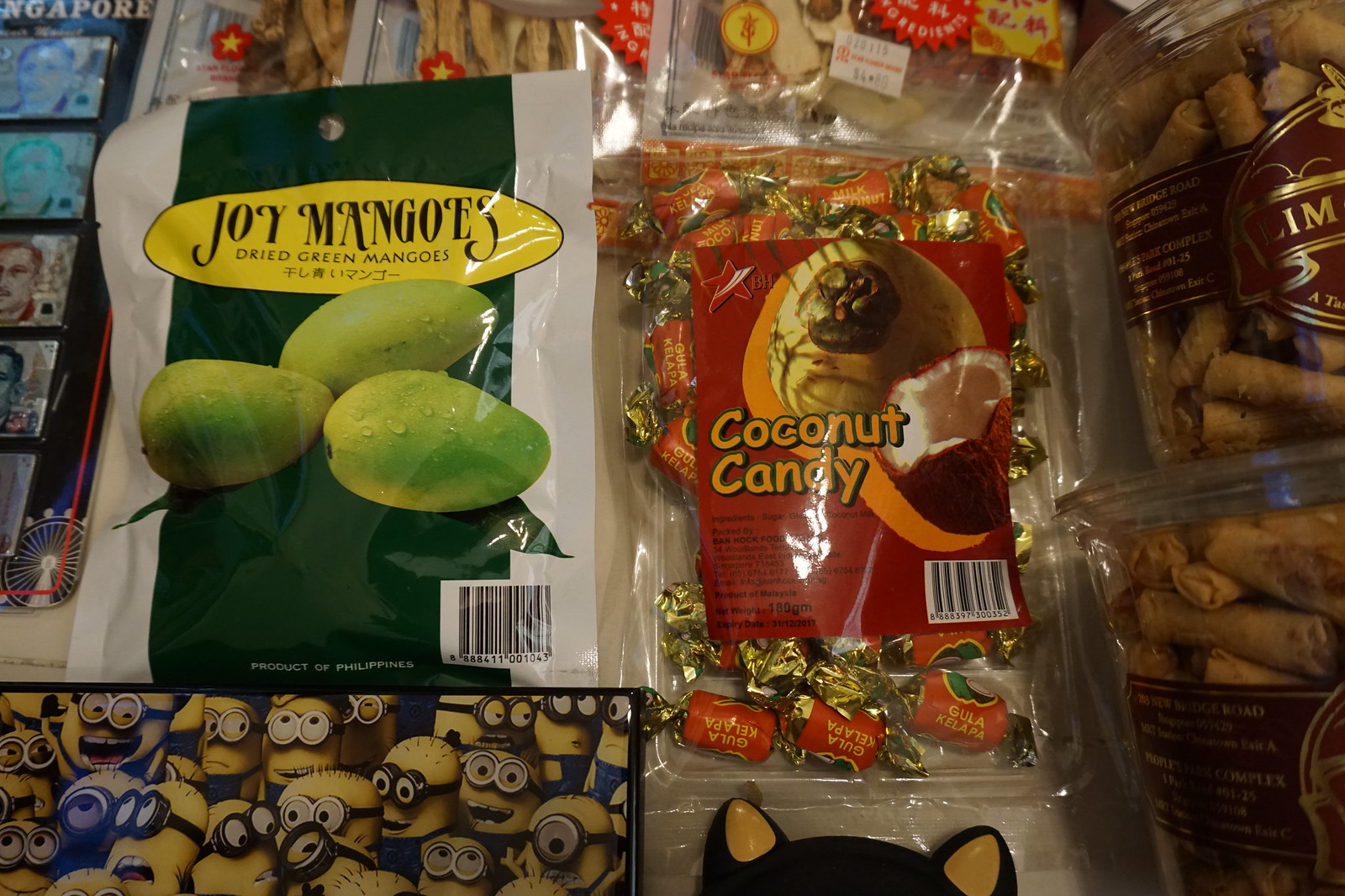The image depicts a seemingly chaotic display of various snacks, likely in a food store, laid out on a table. Centered is a green and white cellophane package labeled "Joy's Mangoes," which contains dried green mangoes and includes Asian characters and the text "Product of Philippines." Positioned to the right is a see-through plastic bag with a red label reading "coconut candy." This bag shows gold-wrapped candies inside, and carries the phrase "Gula Kel Kalapa" along with images of coconuts. Further right are two jars filled with what appear to be elongated, brown candies, though the jars’ labels are partly obscured. On the bottom left of the image, there's a folder featuring Minions with yellow bodies, blue overalls, and black goggles, all staring to the right. The overall color scheme of the items includes yellow, black, various shades of green, gold, red, orange, brown, blue, and light blue. This eclectic assortment of snacks, loosely arranged, suggests a casual and colorful store setting.